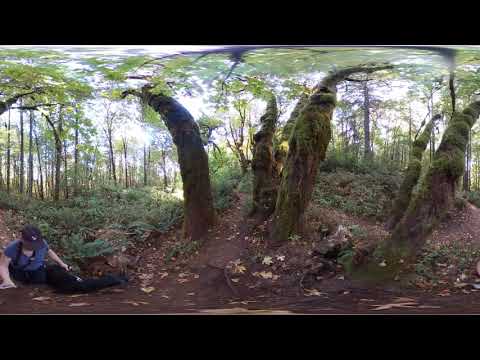A horizontally aligned rectangular photograph with a thick black border at the top and bottom captures a forested area under a clear sky. Various tree trunks, especially noticeable in the middle and right side of the image, rise from the ground and uniquely curve towards the top, possibly due to slight photographic distortion. The trees are mostly leafless on their lower sections, with foliage concentrated higher up. The ground is a mix of soil, dead leaves, and some plant debris, with patches of grass surrounding the tree bases.

Towards the left bottom corner of the image, a person wearing a black cap, black pants, and a short-sleeved blue t-shirt is seated on the dirt among the leaves. The individual appears to be looking down at the ground, possibly searching for something. They have a black strap around their neck, likely holding a camera. The scene is set in an outdoor, daytime environment, characterized by the interplay of browns and greens typical of a wooded area.